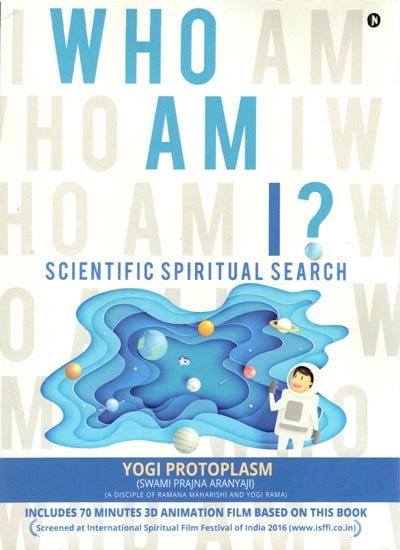The image depicts the cover of a book titled "Who Am I?" with a prominent question mark, where the dot is illustrated as the Earth. The title is written in blue, set against an off-white, creamish background. The eye of the question mark is a darker blue. Repeating across the cover in a light tan font is the phrase "Who Am I?". Below the main title, in blue, it states "Scientific Spiritual Search," written by Yogi Protoplasm, Swami Prajna Aranya, a disciple of Ramana Maharishi and Yogi Rama. The cover includes mention of a 70-minute 3D animation film based on the book, which was screened at the International Spiritual Film Festival of India in 2016, with the website www.isffi.co.in listed twice. The center of the cover features an artistic representation of space resembling a galaxy, complete with various planets, an astronaut figure in a spacesuit, and flowing curvy shapes, all adding to the celestial theme.